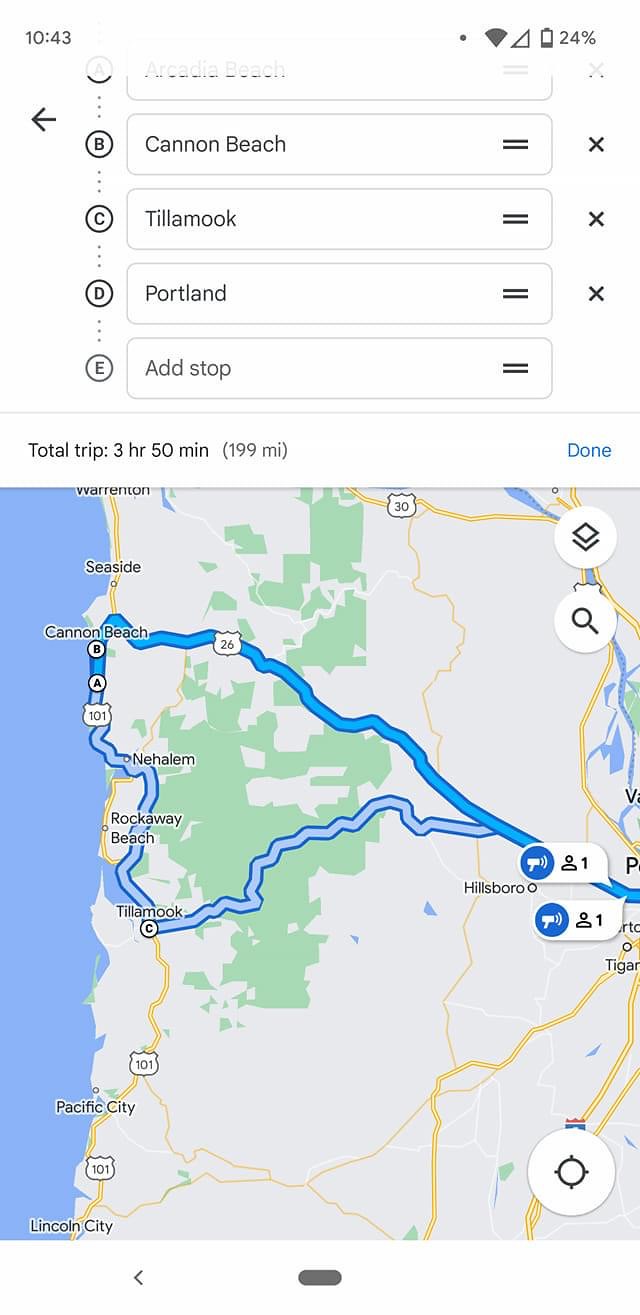This is a detailed, color screenshot from a mobile phone displaying a map application. The top of the image shows the phone's status bar indicating the time as 10:43 a.m., full Wi-Fi signal, no mobile signal (denoted by an empty isosceles triangle), and a battery at 24%. The interface features a series of selectable destinations labeled A through E: Arcadia Beach (A), Cannon Beach (B), Tillamook (C), Portland (D), and Ad Stop (E). Each destination has adjacent lines for further options and an 'X' to remove them. At the bottom of these options, the total trip time and distance are displayed as "3 hours, 50 minutes" and "199 miles."

Below this information, a partial map is visible, primarily highlighting the route in varying shades of blue. The darkest blue marks Highway 26, and the lightest indicates road 101. Key locations like Lincoln City, Pacific City, Seaside, and Warrenton are marked along the coast. The map also shows rivers, possible mountain ranges, and other highways, with green areas likely representing natural landmarks. The map is less detailed than Google Maps, possibly from an off-brand application, and there's an icon resembling a megaphone and person in conversation balloons, though their exact function is unclear. Overall, the map visually guides the user from their location to multiple potential destinations.